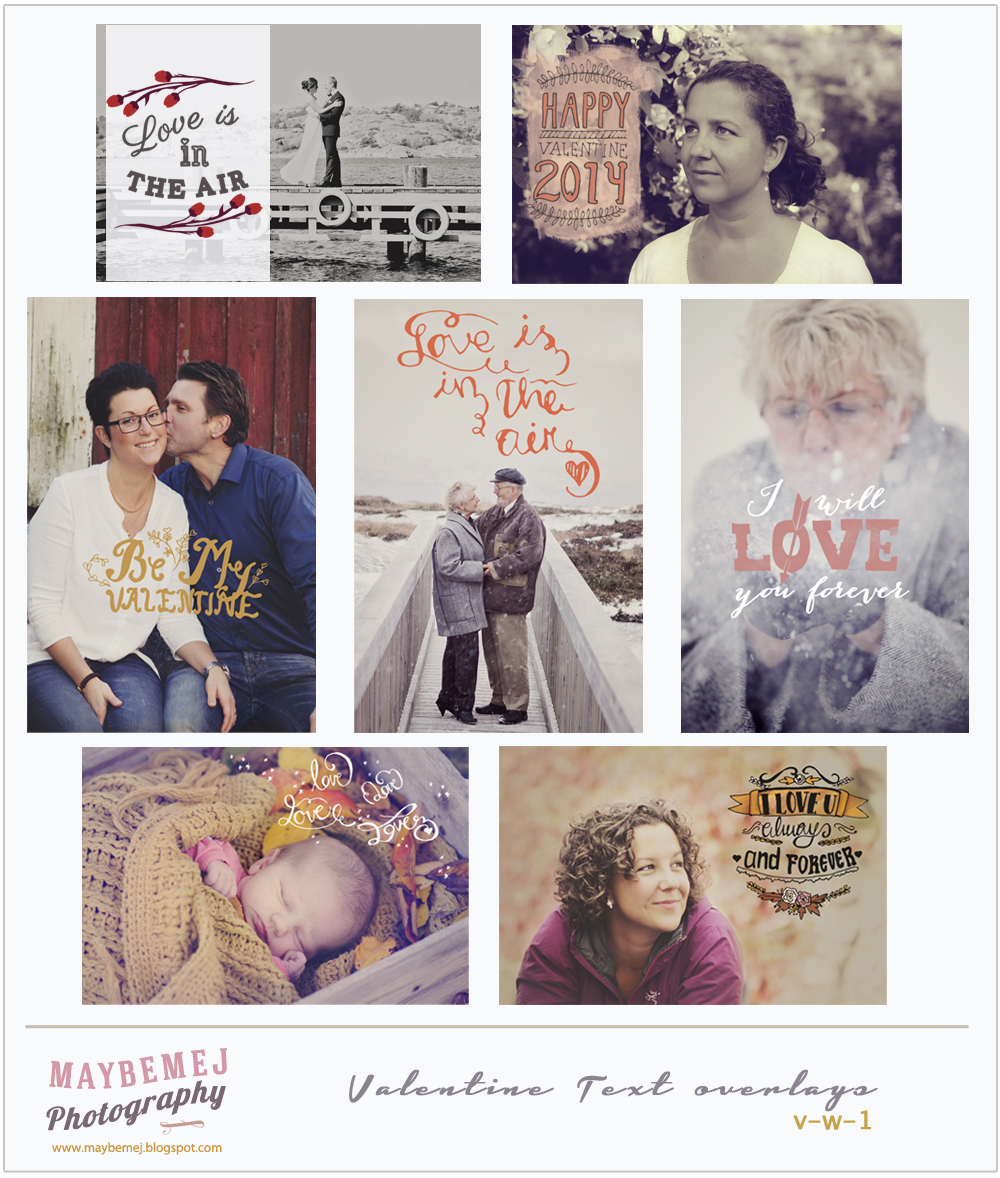In this vertically rectangular advertisement for Maybemnesh Photography, set against a white backdrop with thin gray borders, there are seven distinct photographic images arranged in a grid layout. Each image is accompanied by a romantic text overlay in various styles and colors, fitting the Valentine's theme. 

At the top-left, there's a horizontal picture of a black-and-white photograph showing a bride and groom on a bridge over water with the red text "Love is in the Air." Beside it, another horizontal image features a woman with her hair in a ponytail, wearing a white shirt, and the message "Happy Valentine 2014."

The middle row consists of three vertical rectangles. The leftmost image depicts a man kissing a woman on the cheek, both dressed casually in jeans and t-shirts, with "Be My Valentine" in gold letters. The center image shows an elderly couple embracing on a bridge under the text "Love is in the Air." The rightmost picture in this row features a middle-aged woman blowing bubbles, accompanied by the phrase "I Will Love You Forever."

The bottom row contains two horizontal images. The left picture shows a baby snugly wrapped in a blanket with the caption "Love Love Love." The final image on the lower right depicts a woman with short curly brown hair gazing into the distance, captioned "Love You Always and Forever."

At the very bottom of the advertisement, the text "Maybemnesh Photography" is prominently displayed alongside "Valentine Text Overlays V-W-1" written in cursive.